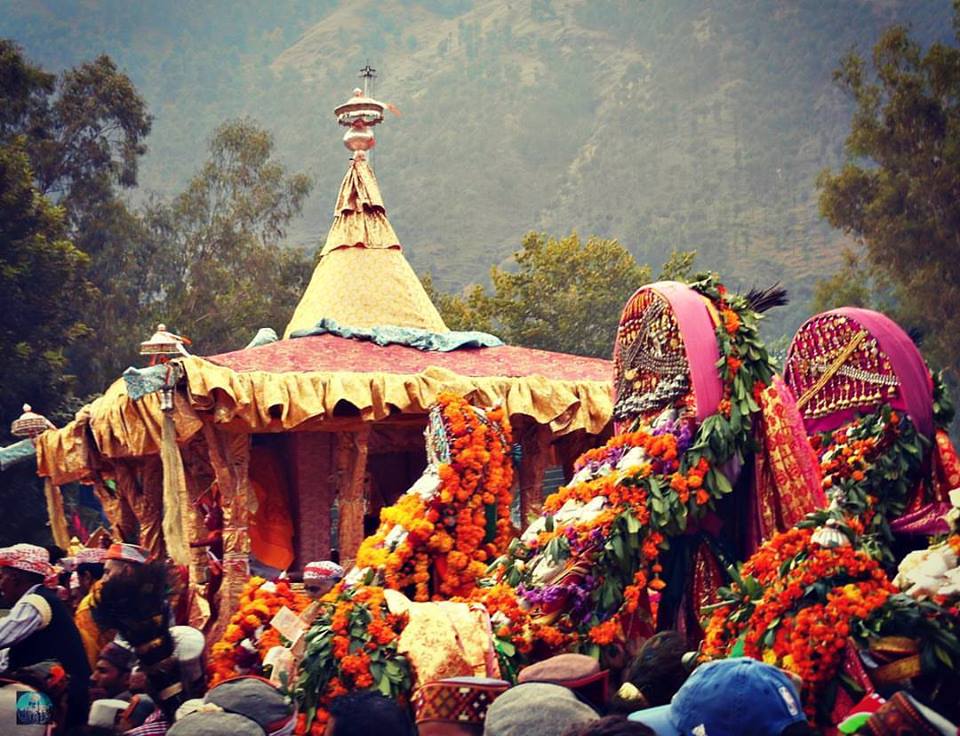The photograph showcases a vibrant outdoor festival set against a scenic backdrop of distant mountains and lush trees. The focal point is a colorful tent-like shelter adorned with an array of bright orange, yellow, and red flowers, with a distinctive cone-shaped top. Surrounding this structure, a lively crowd of people can be seen, many wearing hats, feather boas, and other eclectic attire that adds to the festive atmosphere. Notably, there are decorative items resembling large, rounded statues or flip-flops draped with pink and multicolored flowers at their bases. The scene is filled with vivid colors and floral arrangements, suggesting a celebration or possibly a spiritual gathering, evoking a sense of joyful community spirit.